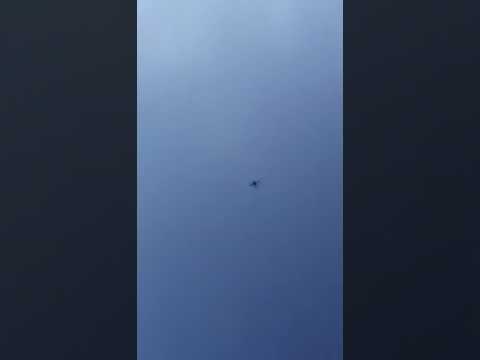The image depicts a vertical 9 by 16 portrait in a light blue color, reminiscent of the sky on a clear day. The central focus of the image is a slightly blurred trio of dots located roughly in the upper third of the blue area. These three dots appear to be floating against the sky-like backdrop, suggesting they could be anything from distant aircraft to small, indeterminate objects such as drones or even insects. This blue center, marked by the enigmatic three dots, is framed on both the left and right by broad vertical black rectangles that border the entire length of the image. These dark vertical bands, which take up a significant portion of the width, give the impression that the blue middle portion is the primary focus, possibly resembling a smartphone screenshot from social media platforms. The absence of any additional elements like clouds or ground further emphasizes the isolated and distant nature of the three blurry spots suspended in the expanse of the blue sky.